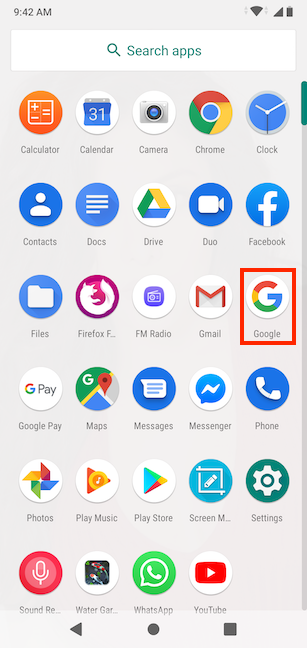This image is a cropped screenshot of a page displaying various Google phone apps. The background is a neutral gray, providing contrast to the elements on the screen. At the top, a large search bar dominates the scene, inviting users to "Search apps" with the text displayed in blue font next to a magnifying glass icon on the left.

Descending from the search bar, the page features multiple rows of app icons arranged in neat rows of five. On the far right side of the image, a small green scroll bar indicates the page is at the top. Each app is positioned in alphabetical order, beginning with the "Calculator" app at the top left corner, followed by "Calendar," "Camera," "Chrome," and "Clock."

Notably, the "Google" app icon stands out in the third row as it is enclosed within a red box, clearly edited onto the screenshot to highlight this specific app. This red box draws the viewer's attention exclusively to the "Google" app, which is the last icon in the third row. The sequence of app icons continues orderly until it concludes with "YouTube," the last icon at the bottom right of the page.

The attention to detail in this arrangement makes the page functional, organized, and easy to navigate, allowing users to quickly find and select the desired app.